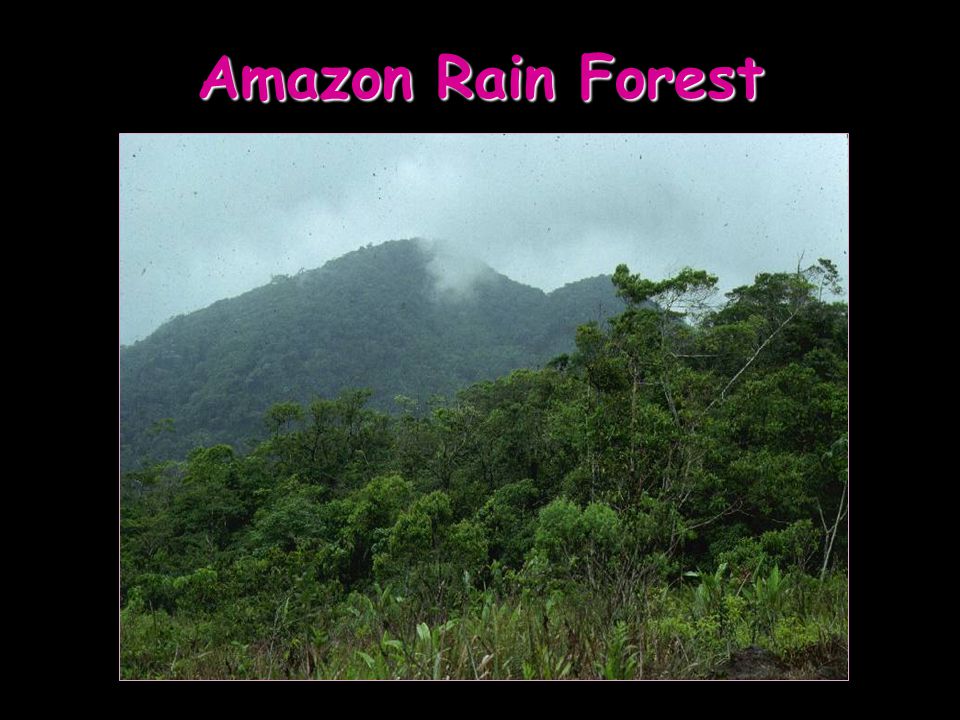The image is a presentation slide featuring a picturesque view of the Amazon rainforest. It has a black background framing the entire slide, with a header at the top displaying the text "Amazon Rainforest" in a rosy pink, Comic Sans-like font, which includes a subtle white shadow for emphasis. The focal point of the slide is a landscape-oriented photograph, slightly lower-centered, depicting the Amazon rainforest. The scene showcases a lush, vibrant green landscape with dense shrubbery and grasses in the foreground. In the background, tree-lined, forested mountains with a dark green hue rise up, partly veiled by white clouds. Smoke can be seen emitting from one of the mountains. The image has a vintage feel, possibly indicated by dots and marks, which could suggest it's an older photograph. The slide’s composition, color scheme, and detail suggest it might be used in a school presentation or a book.